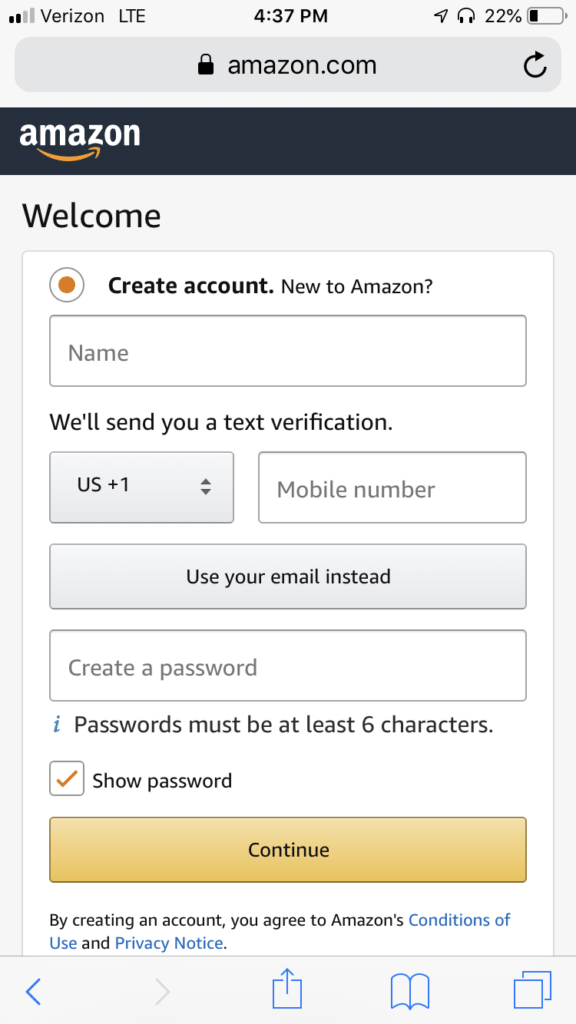The image depicts a webpage for Amazon.com displayed on a smartphone. At the top left corner, the phone shows signal bars along with the text "Verizon LTE". Adjacent to this, at the top right, there's a battery icon indicating 22% charge remaining.

Directly beneath this, there's a gray search bar with black text that reads "Amazon.com". Below the search bar, a black rectangle spans the width of the screen, featuring the white Amazon logo on the left, with the signature orange arrow beneath it.

The main content of the page appears to be a welcome screen for creating a new Amazon account. The header reads "Create account," followed by "New to Amazon?" The form includes several fields for the user to fill out, starting with "Name," accompanied by a note indicating that a text verification will be sent. To the right of this field, there's a box labeled "Mobile number". Alternatively, users can select a gray box with black text that says "Use email instead" to opt for email verification.

Next, there's a white box for creating a password, with the placeholder text noting that "Passwords must be at least six characters". The form concludes with a prominent yellow "Continue" button at the bottom.